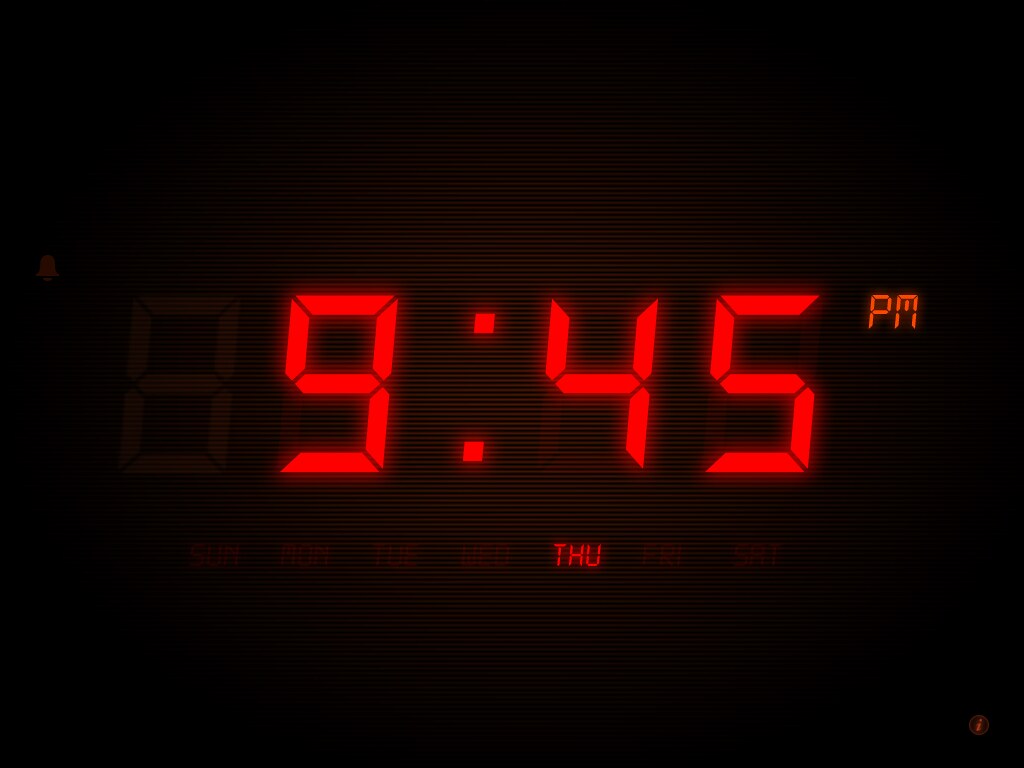The photograph displays a digital clock illuminated against the darkness of night. The clock features bright red, blocky digits reading "9:45 p.m." Below the time, a small red "THU" indicates the day of the week, Thursday. The digit "9" is segmented into six distinct lines, while the "4" comprises four segments, and the "5" is formed by five lines. The abbreviation "p.m." consists of segmented characters, with the letter "M" notably resembling an upside-down "E." The overall scene captures the luminous clarity and segmented structure of the digital display against the surrounding night.